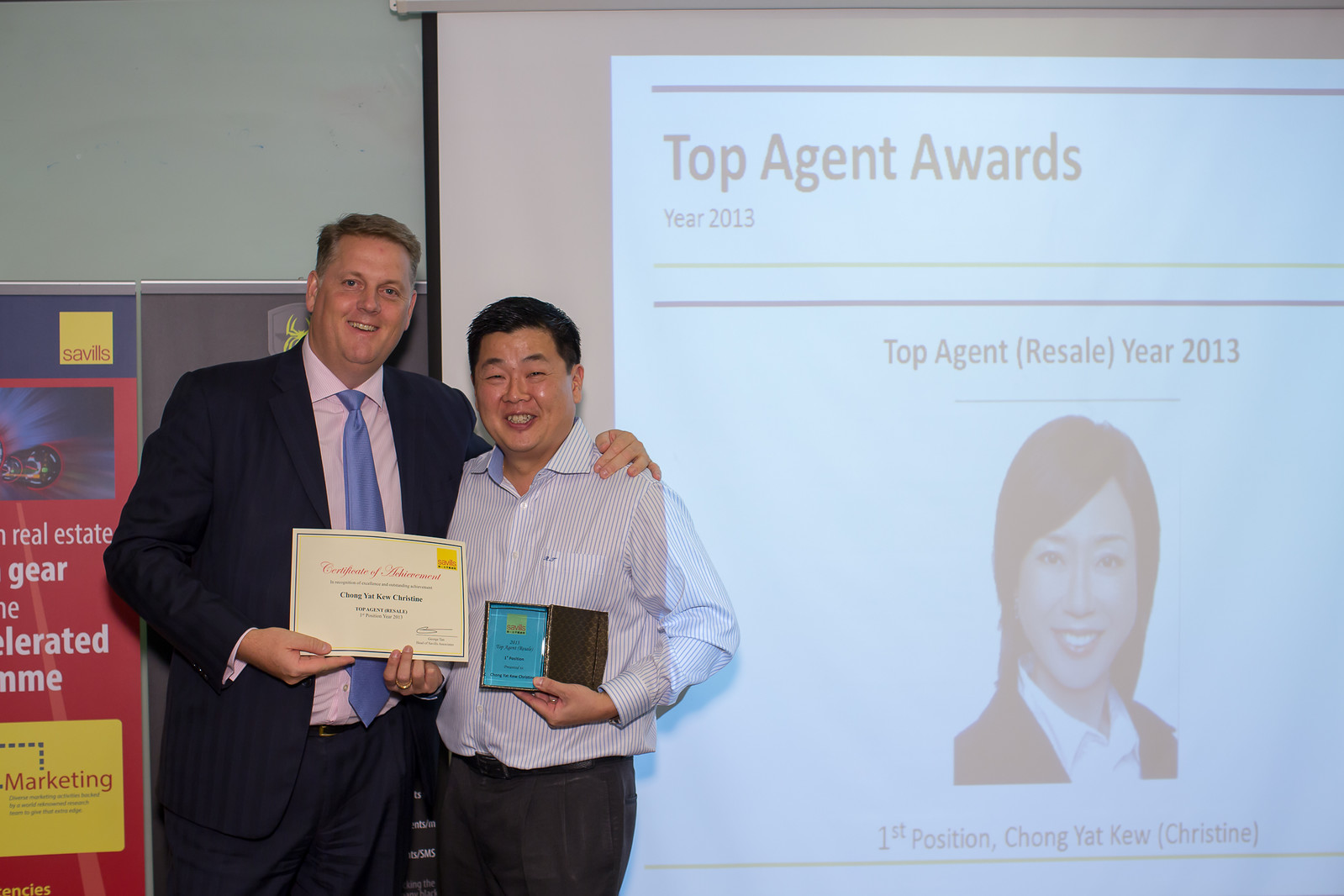The image captures a celebratory moment where two men are standing proudly in front of a projected screen displaying the text "Top Agent Awards Year 2013" and "Top Agent Resale Year 2013." The screen also features the name "Chong Yat Kew, Christine" alongside her photo, recognizing her as the first-position award winner. One man, wearing a striped white and blue shirt with black pants, holds a certificate of excellence in one hand and a leather-bound award in the other. This man appears to be Asian and is smiling. Beside him stands a taller, heavier-set Caucasian man dressed in a blue business suit with a pink shirt and blue tie, possibly his boss, who is also smiling. Both men are clearly celebrating the achievement. The background includes a partial view of a real estate advertisement with some yellow and red elements on the left wall, adding context to the professional setting. The main colors in the image are gray, blue, red, and yellow.